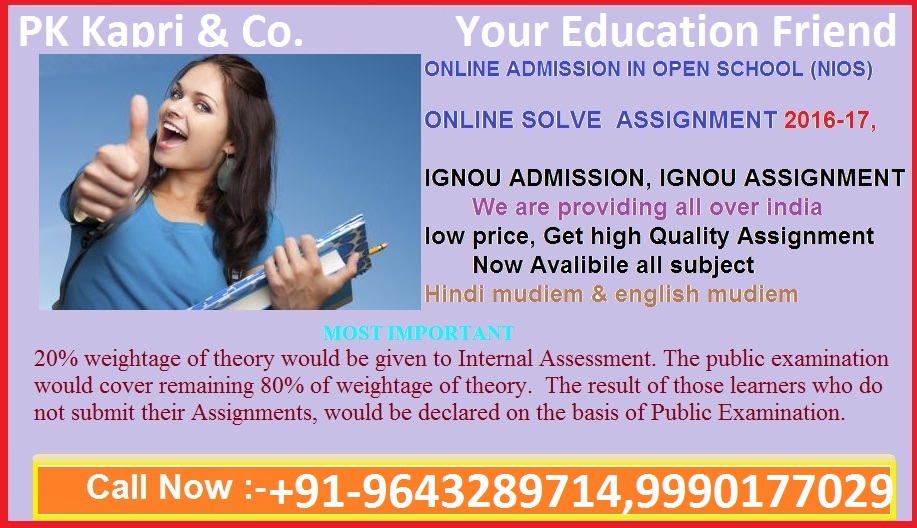A young girl, dressed in a blue shirt, gives a thumbs up with a bright smile on her face while holding a stack of books in her left hand. She serves as the cheerful mascot for Capri and Co, your dedicated educational companion. This service offers online admissions and open schooling across India, providing high-quality assignments at an affordable price. Their comprehensive offerings include assignments for the academic year 2016-17, such as the IGNOW admissions and assignments, available in subjects like Hindi, MUDLEM, and English MUDLEM. Notably, 20% of the theory weightage is assigned to internal assessments, while the public examination covers the remaining 80%. For those who fail to submit their assignments, their results will be determined solely by the public examination. For more information and to avail these educational resources, call +91-9643289714, 9999077029.